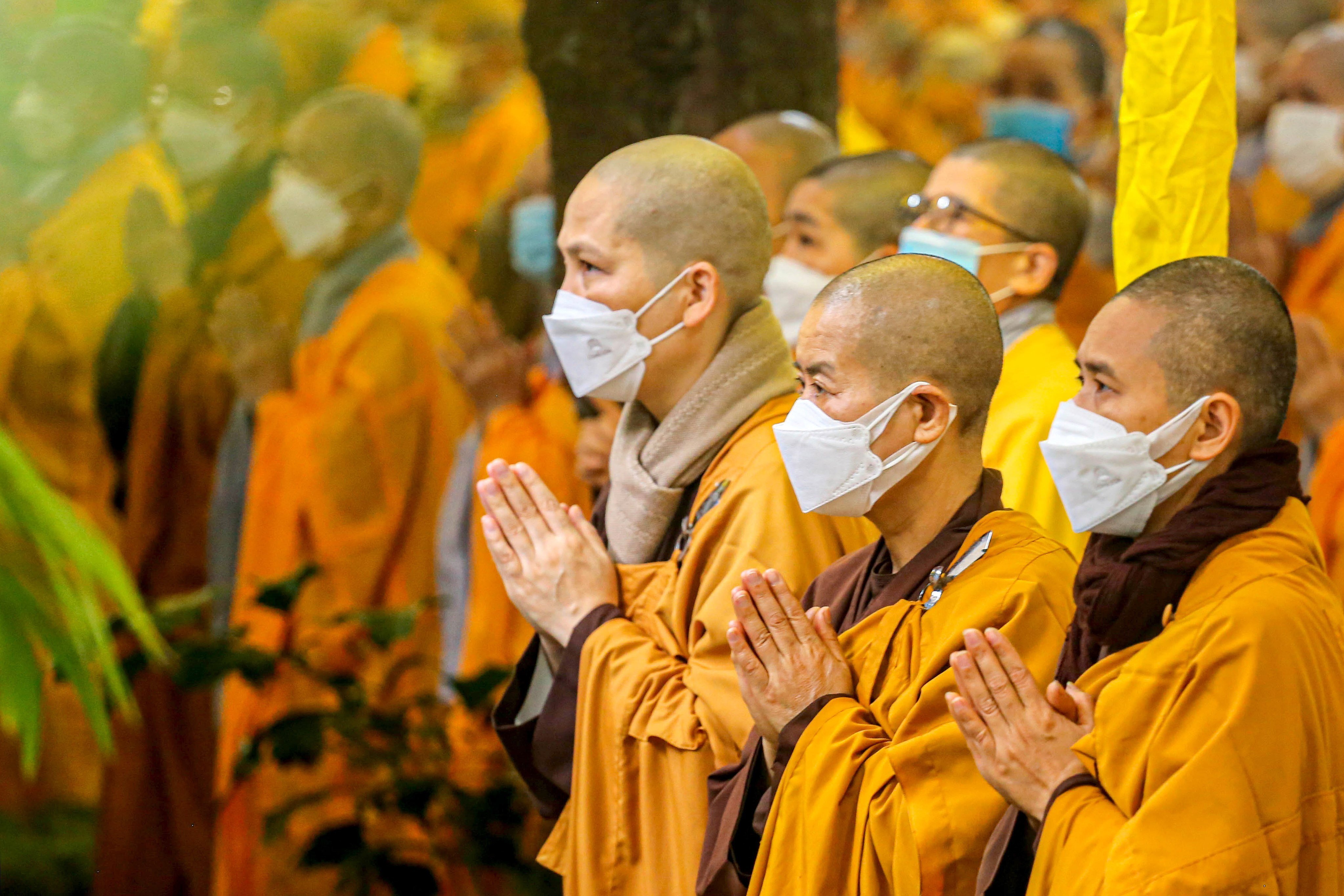In the image, a congregation of Tibetan monks is depicted in an atmosphere suffused with a yellowish hue. The foreground features three monks clearly in focus, their shaved heads adorned with a bit of stubble. These monks wear yellow robes and have their hands clasped in prayer. Among them, two are distinguishable by their dark brown scarves, while another dons a light brown one. All monks in this scene are wearing masks, indicative of the COVID-19 pandemic precautions.

In the blurred background, more monks are discernible, adding to the sense of a vast assembly. Some background monks are notable for their colorful scarves—gray and black being prominent among them—a few wearing glasses. They are all similarly garbed in yellow robes with occasional red accents, and all monks have their hands clasped in prayer. There is a patch of greenery visible to the left, adding a natural element to the setting. The monks uniformly face left, deep in their contemplative practice.